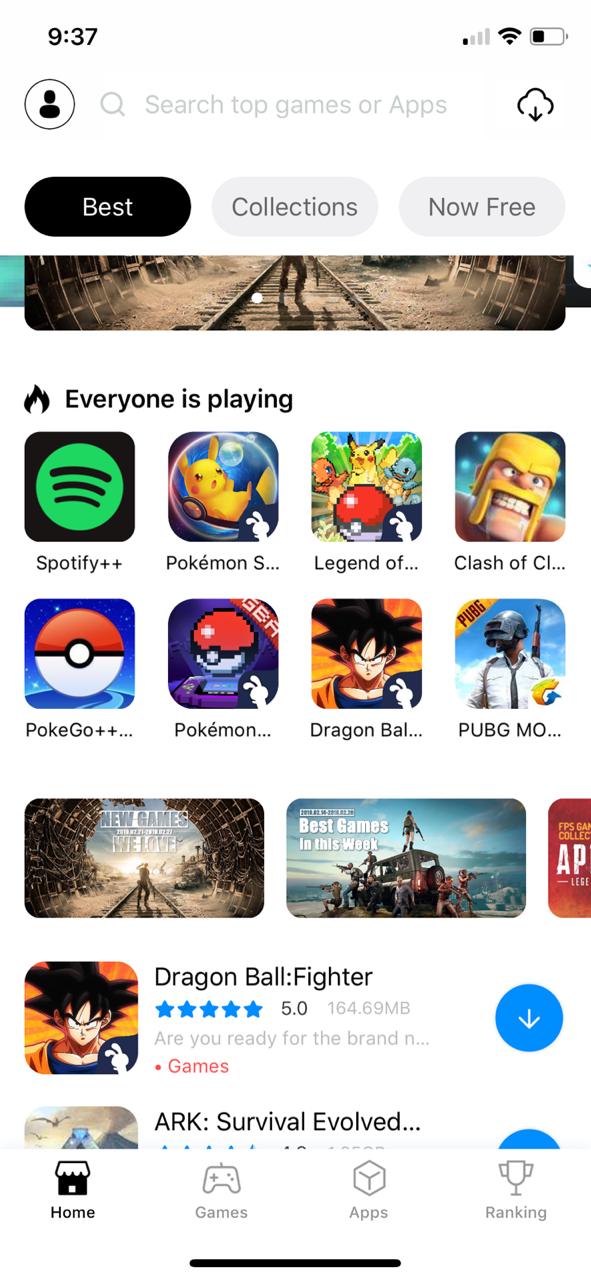The image depicts a smartphone screen displaying an app store interface. 

At the top right corner, the time reads "9:37", accompanied by a Wi-Fi signal icon and a battery indicator showing a nearly full battery within a circular icon. Just below, there is a search bar marked by a magnifying glass.

The main section of the screen shows a series of app categories and featured items:

- A "Switch Top Games or Apps" section with a cloud icon featuring a downward arrow indicating downloadable content.
- A black circle with white text labeled "Best".
- A prominent gray oval in the center labeled "Collections" and another gray oval reading "Now Free".

Featured apps and content are visually diverse:

- An image depicting a brown background and a railroad.
- An area labeled "Everyone is Playing" accompanied by fire graphics.
- A black square with a green circle labeled "Spotify Plus Plus".
- Various Pokemon characters are visible: Pikachu, Charmander, and Squirtle, alongside a section titled "Legend of Something".
- An app area labeled "Pokemon Plus Plus" featuring Pokemon graphics at both the top and bottom.

Lastly, at the bottom of the screen, there are categories titled "Games", "Apps", and "Ranking".

Overall, this is a detailed snapshot of a smartphone app store interface offering numerous apps and detailed visual cues.